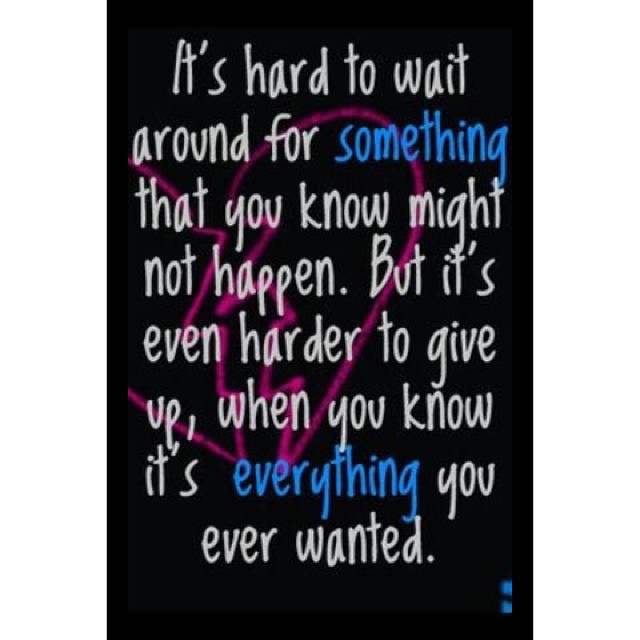The poster is a black rectangular illustration in portrait orientation with the vertical sides longer than the horizontal sides. The background features a solid black color with an abstract pink sketch that resembles either a squiggly line, a Pac-Man ghost, or a heart with a break in the center. Overlaying this background is a handwritten font in white that covers the entire image from top to bottom, reading: "It's hard to wait around for something that you know might not happen, but it's even harder to give up when you know it's everything you ever wanted." Key words "something" and "everything" are highlighted in light blue. Additionally, the bottom right corner of the poster has two small blue dots. The overall design combines elements of graphic design and typography.